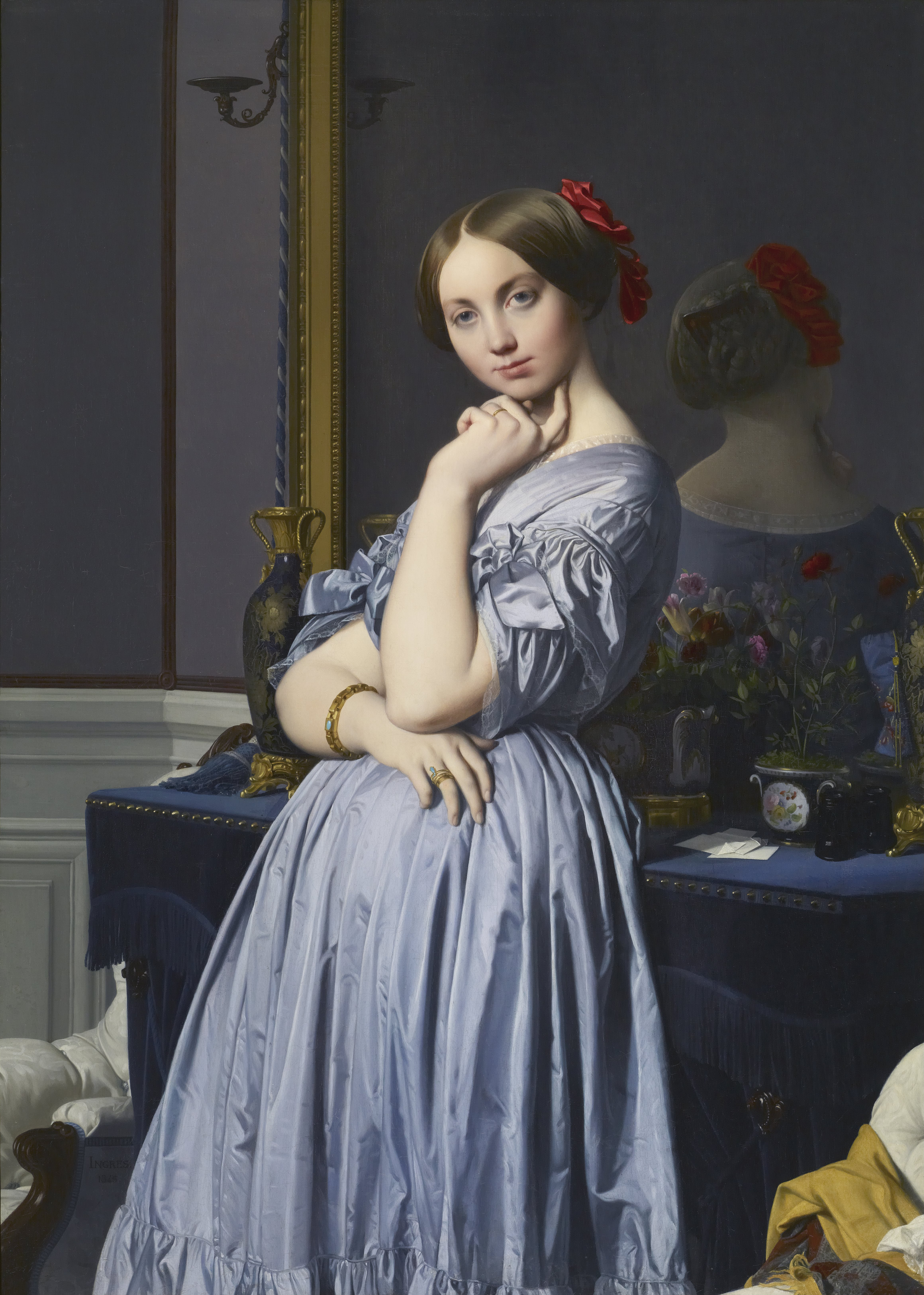This stunning self-portrait captures a moment of introspective beauty, featuring a woman illuminated against a dark backdrop. Seated centrally within the frame, she gazes thoughtfully towards the viewer, dressed in a long, blue silk or satin dress adorned with ruffles around the sleeves and hem. Her hair is elegantly styled, accented by a red rose or ribbon. One arm is gracefully crossed at her waist, while the other is bent, with her hand resting under her chin, adding a contemplative touch to her pose. A bracelet gleams on her wrist, adding a delicate detail to her outfit. 

The setting evokes a sense of timeless elegance, reminiscent of classical 1700s portraiture. Behind her stands a large wooden dresser with an attached mirror, reflecting her shadow and adding depth to the scene. The dresser top is decorated with a vase, flowers, and assorted small items, lending a lived-in, intimate feel to the space. The surrounding colors of tan, brown, white, gold, red, olive, and yellow harmonize to create a rich, textured environment. The wall behind her features a gray upper half and white wood molding, further enhancing the classical ambiance of the portrait.